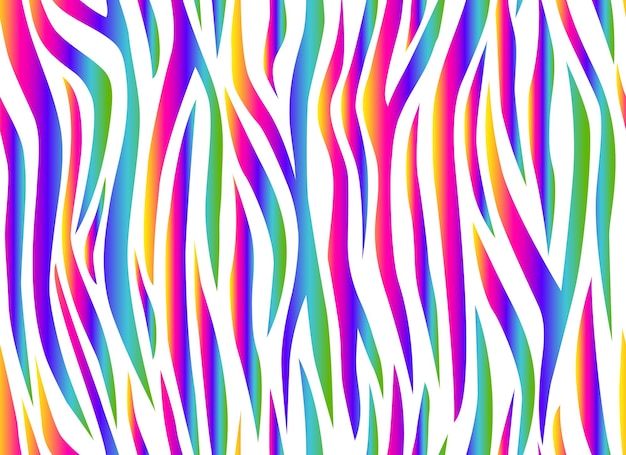The image presents a captivating pattern of vibrant, tiger-striped lines against a pristine white background, reminiscent of zebra stripes with a colorful twist. These stripes are far from uniform; they curl and curve, interlacing and varying in thickness as they extend fully to the edges of the image. The larger stripes prominently feature shades of dark blue, purple, and pink, seamlessly transitioning into bright orange and a touch of yellow. Interspersed among these are smaller stripes and edges displaying vivid greens. The colors blend beautifully, creating a gradient effect that suggests a dynamic, digital artistry. The overall effect is a striking rainbow rendition of zebra stripes, possibly suited for use as a digital background or piece of digital art.